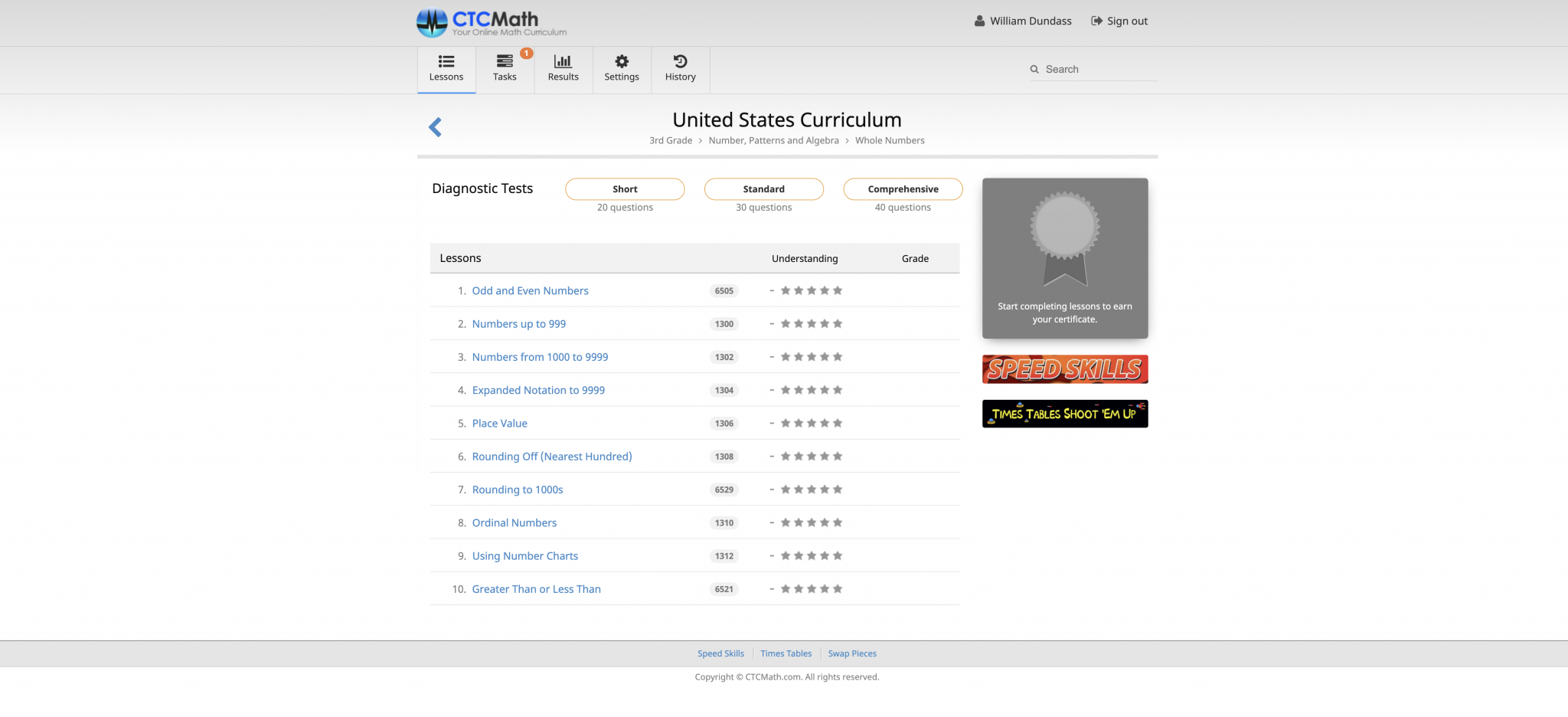The image displays the interface of the CTCMath website. The CTCMath logo, a circle with a prominent black 'M' in the center, is positioned to the left side of the header. On the right side of the header, a user named William Dundas is logged in, with a visible 'Sign Out' button to logout from the website.

Below the header, on the left-hand side, there is a vertical menu featuring various icons and labels for different sections: Lessons, Tasks, Results, Settings, and History; each accompanied by illustrative icons.

Dominating the center of the screen is a heading in large bold font that reads "United States Curriculum." Below, on the left-hand side, there is another heading titled "Diagnostic Tests." This section includes a series of buttons labeled 'Short,' 'Standard,' and 'Comprehensive,' each corresponding to different lengths of diagnostic tests with varying numbers of questions.

Below the 'Diagnostic Tests' section, a list of lessons is displayed. Each lesson title appears as a blue hyperlink, suggesting they are clickable for more information or content. Adjacent to each lesson title are numerical indicators and star rating icons. Currently, none of the lessons have star ratings assigned, but the placeholder suggests future ratings may be available.